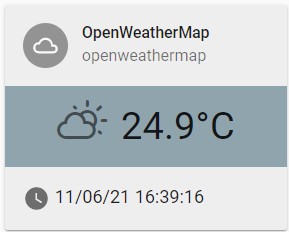The image displays a small user interface panel on a computer screen with distinct sections and icons. At the very top, there is a light grey border. On the left side, there's a dark grey circle featuring a small, white-outlined cloud. To its right, a header reads "OpenWeatherMap" in black text, with each word's initial letter capitalized. Directly below it, there is the same text, "openweathermap," but in a lighter shade of grey and entirely in lowercase. 

Beneath these labels, a darker grey panel showcases a small cloud icon next to a sun on the left side. Beside this icon, the current temperature is prominently displayed as "24.9°C" in much larger font. 

Further down, another light grey panel, identical to the top border, is visible. On the left side of this panel, there is a grey clock icon showing approximately 4 o'clock. The clock is accompanied by numbers: 11, 06, 21, 16, 39, 16. This concise yet informative panel provides a quick visual summary of the weather and time information.